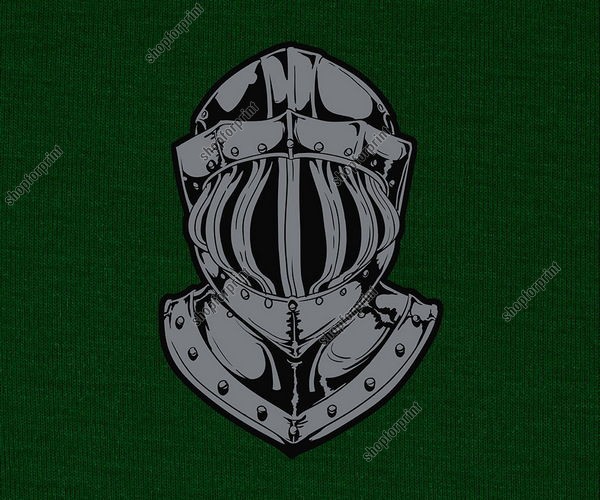This is an image printed on a dark green fabric, which appears to be a t-shirt or sweatshirt. The backdrop's textured detail suggests it's either of these types of clothing. The central illustration is of a knight's helmet, facing forward, illustrated in shades of black and gray. The helmet showcases intricate details such as rivets along the forehead and neck, where the armor pieces join. The visor area, where one would see out of, is depicted in black. The words "SHOP TO PAINT," also rendered in a dark green with a white outline, are repeated thrice across the image: in the lower left-hand corner, the upper left-hand corner, and the bottom right-hand corner towards the center. This watermarking suggests the image is from "Shop to Paint," highlighting their branding. The overall depiction combines the starkness of medieval armor with a modern design element, making it a striking print for apparel.